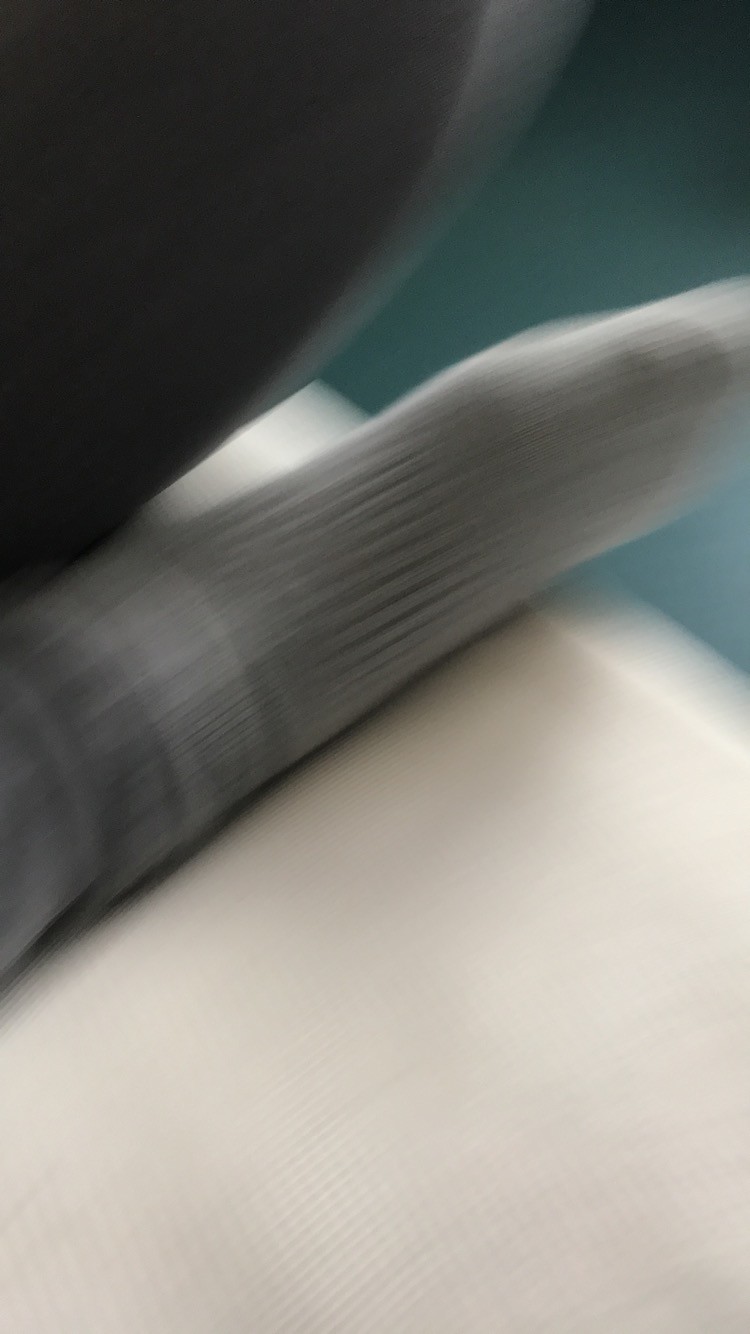The image is notably tall and suffers from poor quality, being blurry, fuzzy, and pixelated. Central to the composition is a long, blurry, gray object positioned on a white platform. Additionally, there is a black block located in the upper left corner, while the upper right corner features a dark green block. The low resolution and significant blurriness make it challenging to discern precise details of the scene.